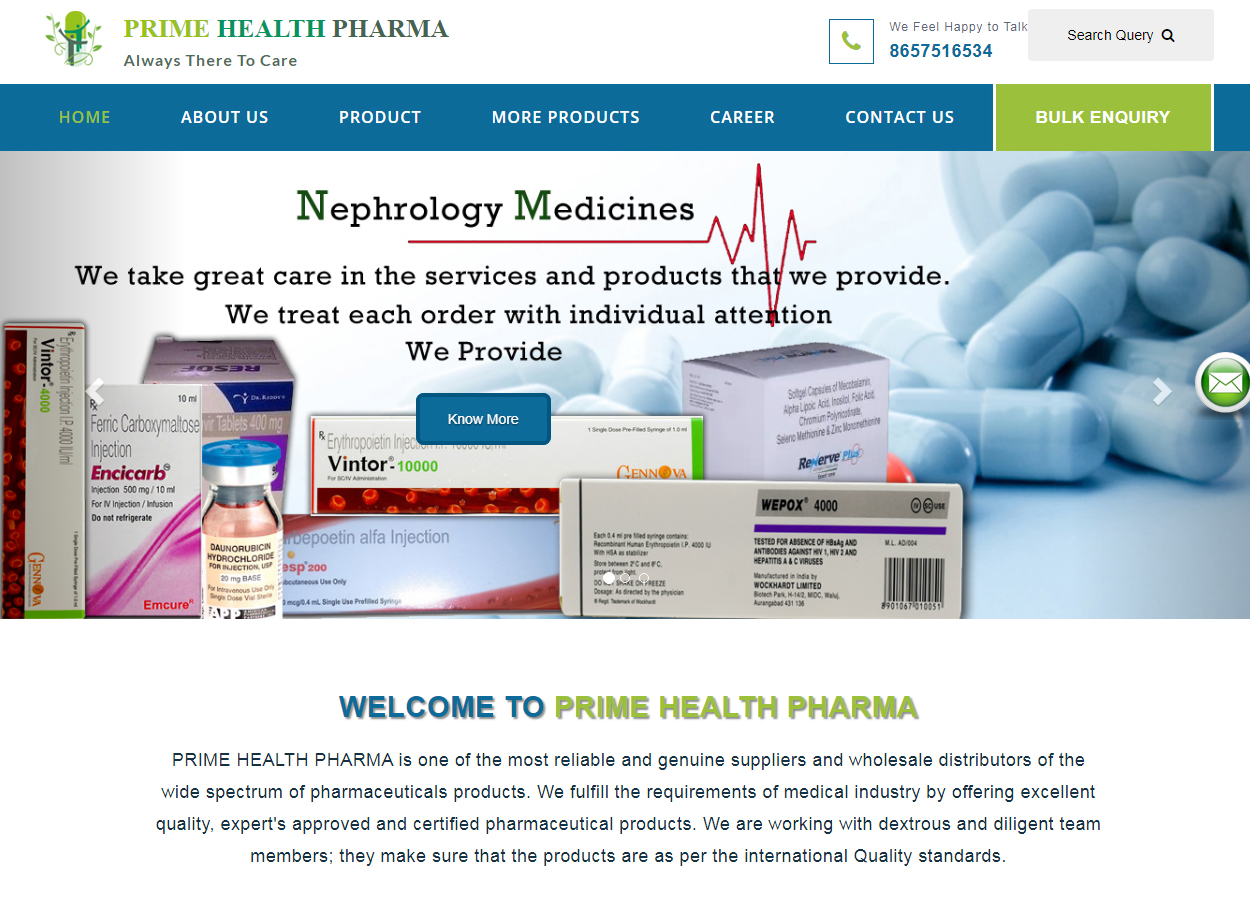The home page for Prime Health Pharma is thoughtfully designed, featuring a prominently placed logo on the left side. This logo is minimalistic and rendered in green, vaguely resembling a tree. Along the top of the page, a navigation bar with a blue background provides links to Home, About Us, Products, More Products, Career, and Contact Us. One distinct section labeled Bulk Inquiry stands out with a green background.

On the top right of the page, there is a clearly visible phone number for inquiries and a search bar for navigation. The centerpiece of the homepage is a main image related to Nephrology Medicines, accompanied by the text: "We take great care of the services and products that we provide." This section showcases various medications, including Ventor and NCICARB, although their specific uses are not detailed.

At the bottom of the page, a welcoming message introduces Prime Health Pharma as one of the most reliable and genuine suppliers and wholesale distributors. The page is designed to be interactive, allowing users to scroll horizontally to access additional articles and features about the company and its offerings.